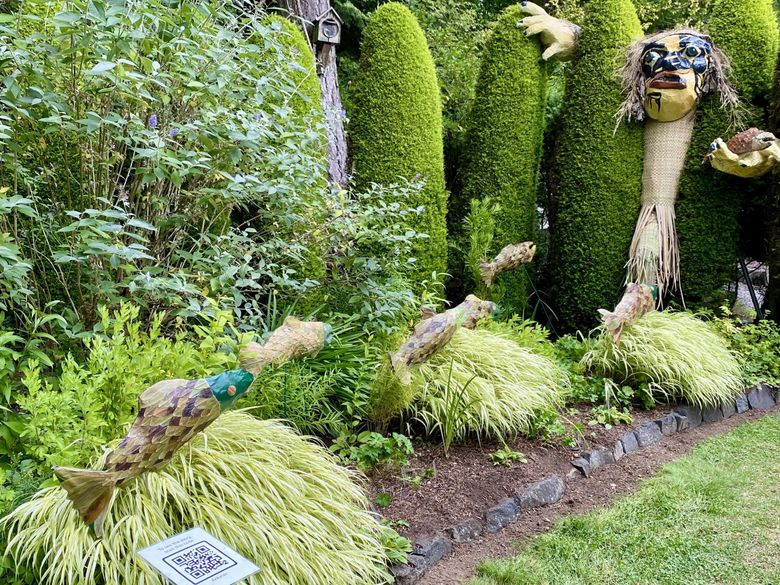The image captures a meticulously maintained garden with an assortment of greenery and whimsical decorations. Dominating the scene are three large, oval-shaped shrubs that are solid green, reminiscent of elongated cucumbers or cacti. These shrubs stand out against a backdrop of lush, leafy plants including hosta and a few patches of green grass on the bottom right. The garden's ground is covered with brown dirt and some mulch, bordered neatly by gray rocks.

Amongst the greenery are several ornamental features. On one of the shrubs leans a striking scarecrow figure with a painted face. This figure exhibits a vibrant yellow complexion with contrasting blue and black detailing, large red lips, and wheat stalk-like hair, giving it a quirky appearance. The scarecrow's hands, painted yellow, are prominently displayed, with one seemingly holding an indistinct object that could be a fish or fruit. Additionally, the garden is adorned with smaller puppet-like ornaments in the shape of fish, each featuring a teal blue face with burgundy and yellow triangular designs on their backs, appearing as though they are swimming towards the scarecrow.

To the left of the scene are dense clusters of leaves and leafy flowers, adding to the garden’s lush ambiance. Nestled within the plants is a whimsical outdoor ornament resembling a yellow and blue mask, with an accompanying QR code plaque, inviting further interaction or information. This captivating tableau combines natural beauty with playful artistry, creating a unique and detailed garden display.